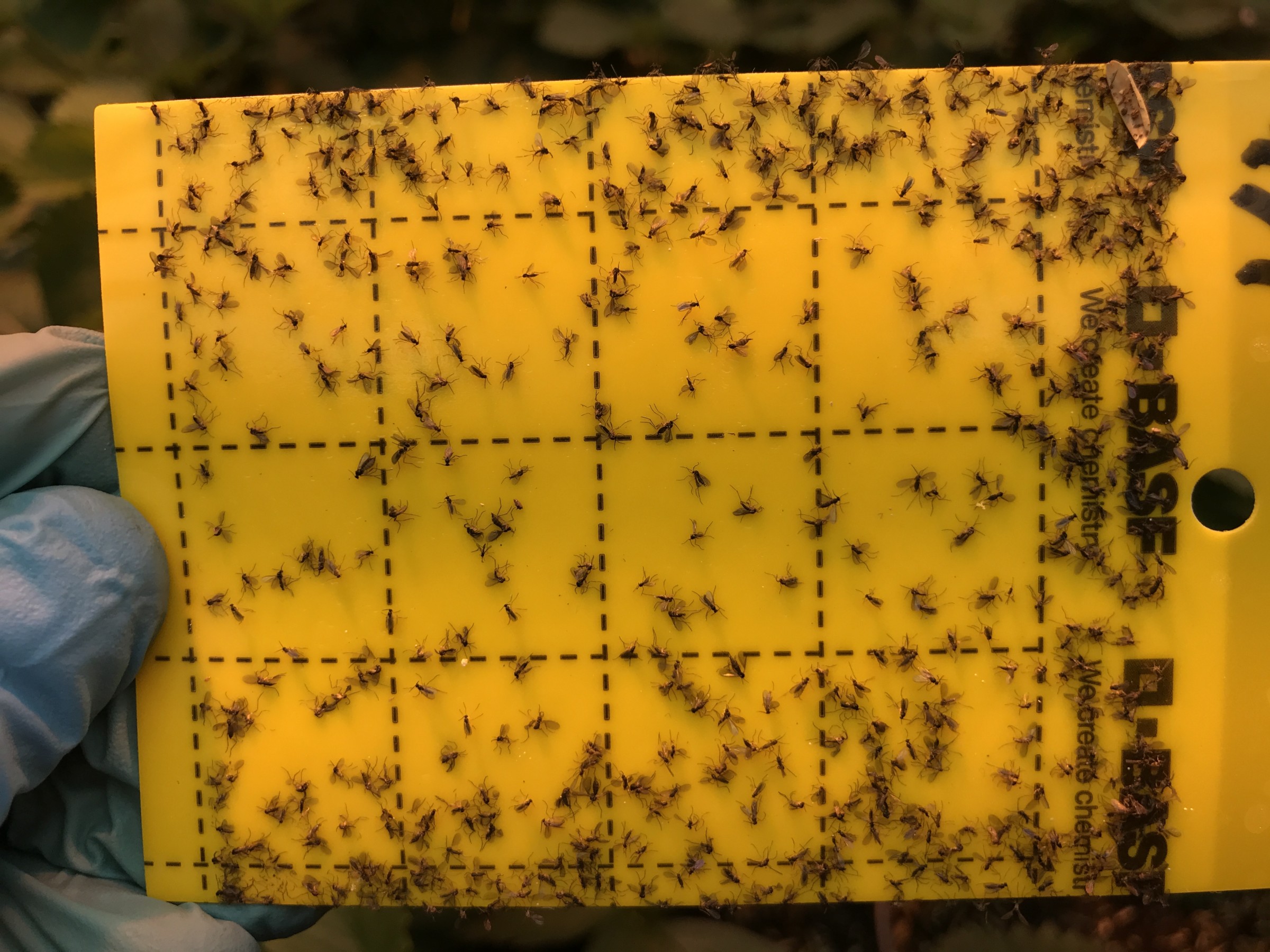This large square image is a close-up of a yellow, rectangular sticky trap, likely made of plastic and covered in countless tiny brown ants. The trap, held sideways, features a small hole in the center-right and is marked with the faint and partially obscured text "D base" or possibly "B.A.F.F.," followed by "we create Chemistry." The quadrants are defined by dotted lines, with 12 visible squares that extend further beyond the image's frame. The trap is densely populated with ants, primarily clustering around the outer edges, while the center area remains relatively less crowded. A person's gloved hand, appearing on the left side and clad in a gray rubber glove, holds the trap, emphasizing the object's role in pest control.